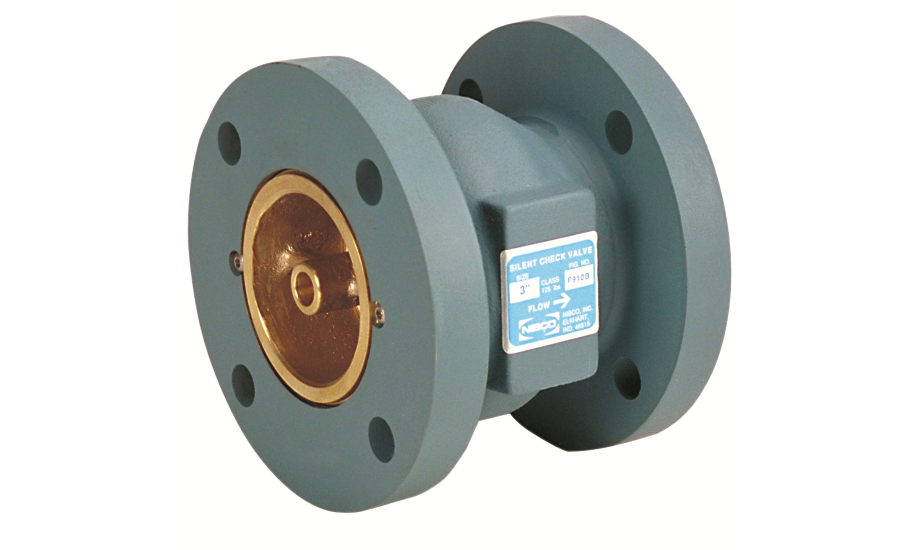This photograph features a mechanical component known as a "silent check valve," prominently displaying this label along with the specifications "3 inches," "Class 125," and "Figure No. F9100." The equipment is primarily a grayish teal or mint green color, made of metal, with two disc-shaped ends, each containing four holes likely for assembly or mounting purposes. These discs are connected by a bulging central tube. At the center of the valve, there is a distinctive gold circular element resembling a bowl with a central pipe protruding from it. Additional markings include an arrow indicating the direction of flow towards the right and the manufacturer's name, NBCO, amongst other less legible details. This piece of equipment is designed to be both functional and structurally integral to a larger mechanical system.